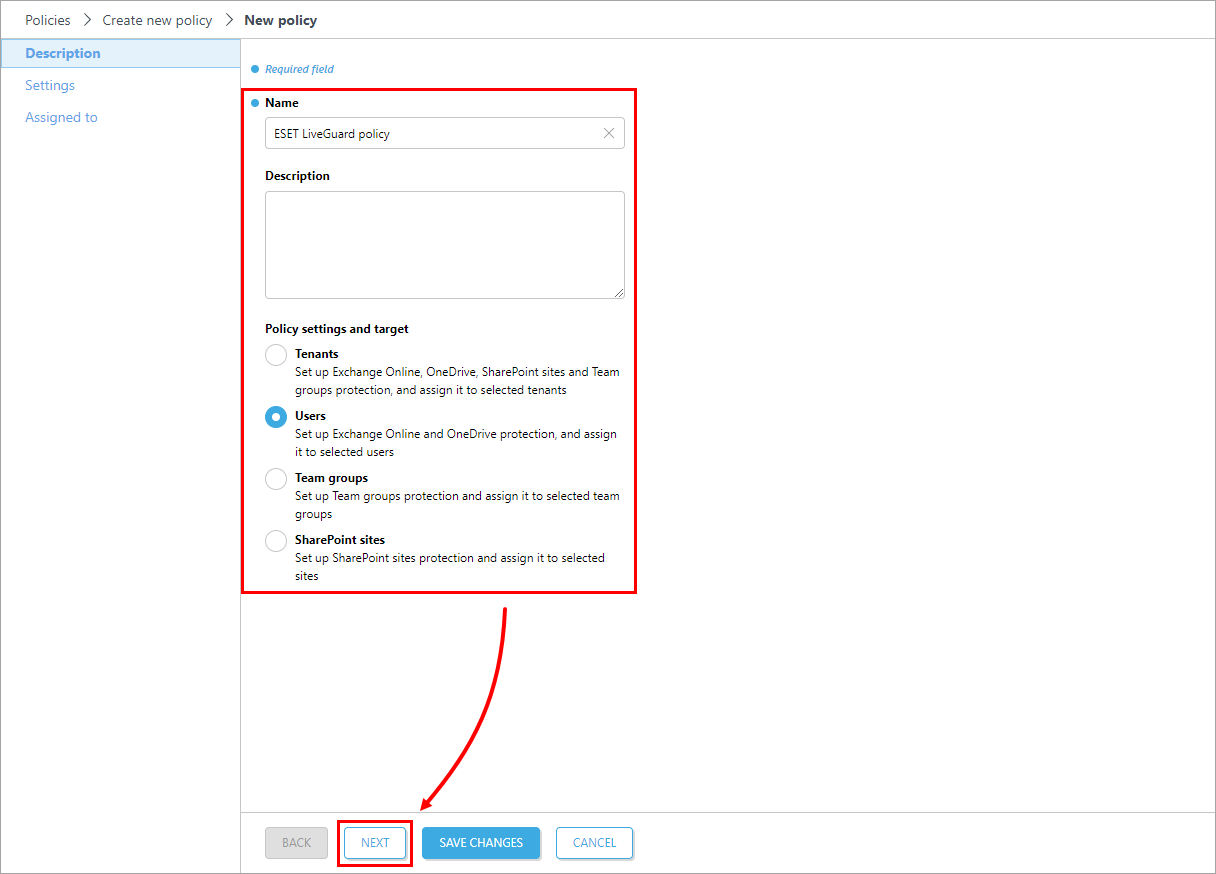The image depicts a user interface screen for creating a new ESET LiveGuard policy. At the top, the title "Policy: Create New Policy" is displayed, with the "New Policy" section highlighted in black. Below, the word "Description" appears in blue. Adjacent to it, there are tabs labeled "Settings" and "Assigned To".

On the right side, there's a designated "Required Field" marked with a blue dot, prompting the user to input a "Name," which also has a blue dot. The name field is filled in with "ESET LiveGuard Policy." The "Description" box is currently blank.

Further down, various policy setting options and target assignments are listed:
- **Tenants**: Configure protection for Exchange Online, OneDrive, SharePoint sites, and team groups, and assign it to selected tenants.
- **Users**: Configure protection for Exchange Online and OneDrive, and assign it to specific users.
- **Team Groups**: Configure protection for team groups and assign it to chosen groups.
- **SharePoint Sites**: Configure protection for SharePoint sites and assign it to selected sites.

A red arrow points to a "Next" button, which is highlighted in a red box. To its left, the "Back" button is displayed in black, while on the right side, a "Save Changes" button appears in blue, and a "Cancel" button is also present.